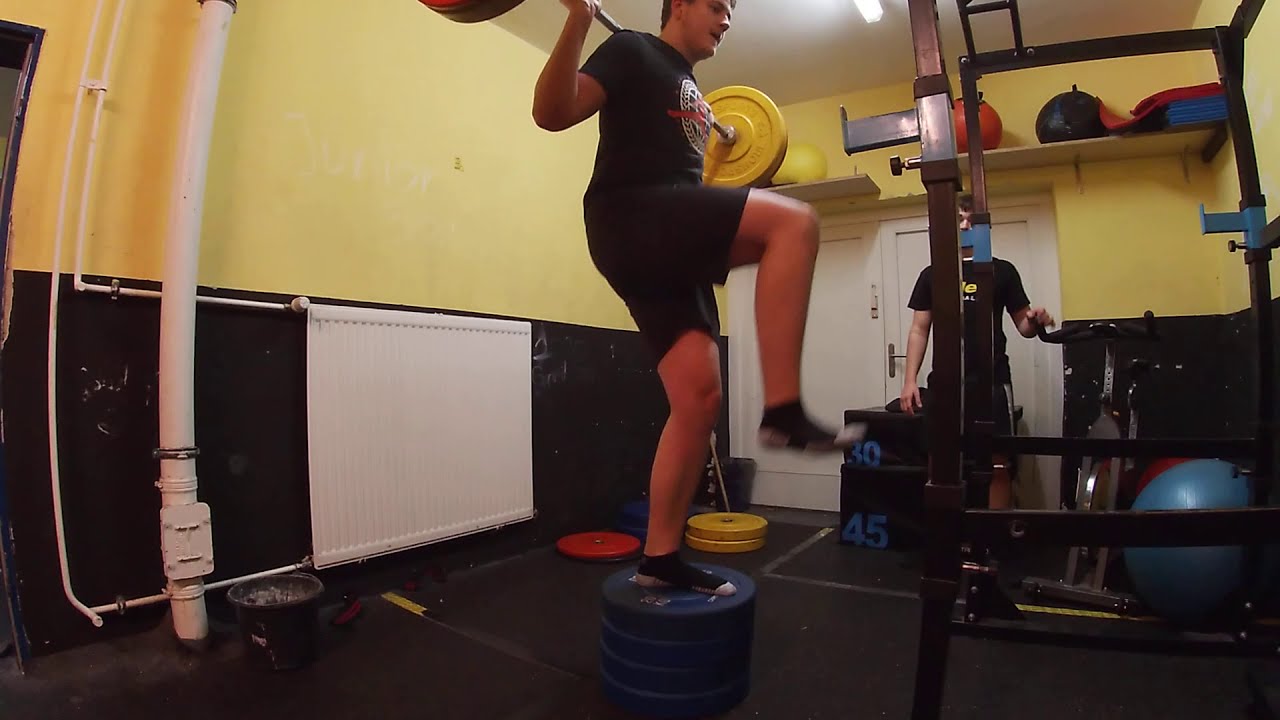In this image, we observe a young Caucasian man working out in a gym environment. He is poised on his left foot atop a stack of four large blue dumbbell weights, which serve as his platform. His right knee is elevated, suggesting he is either in the midst of a one-legged squat or balancing, as the motion blur indicates movement. Clad entirely in black—shorts, t-shirt with a logo, and short socks—he holds a heavily loaded barbell across his shoulders with several 45-pound plates on each side.

The gym itself features distinctive decor: the upper half of the walls is painted yellow, while the bottom half is black and white. The floor is covered with scattered weights, and a blue exercise ball is tucked into the lower right corner. A black squat rack stands directly in front of him, complete with metal structures and various gym equipment around.

In the background, partially obscured by the squat rack, stands another young man dressed in black shorts and a black shirt. His face is hidden by the white bench he is behind, and he appears to be observing the workout. Behind him is a door painted white, along with a shelf holding miscellaneous gym objects. The room's constricted feel is accentuated by the wall piping visible on the left side.